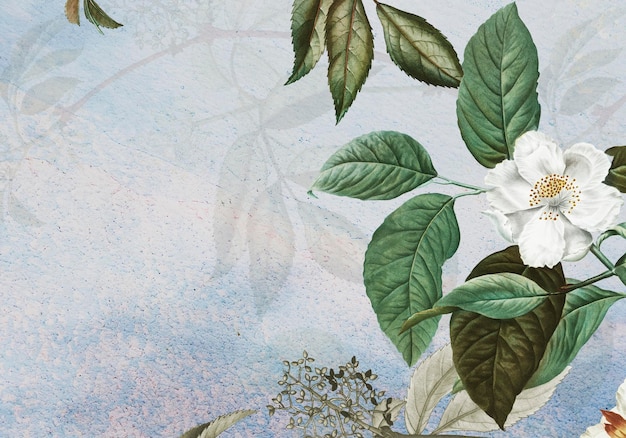This image is a detailed depiction of a white flower with a yellow center, surrounded by an assortment of green leaves varying from dark to light hues, some even with a feather-like appearance. The focal point of the image is a clear blue puddle of water reflecting both the white flower and a cluster of dark green leaves above it. Complementing the rich, vivid colors of the foliage, the background features a textured interplay of light blue, white, and subtle hints of pink, creating a soft, dappled effect. Additionally, there's an area with orange against the white backdrop on the lower right side, adding a touch of warmth to the overall composition. The entire scene appears as a rendering that could be a photograph of a drawing or a digitally rendered graphic, and it exudes a harmonious blend of natural and artistic elements.